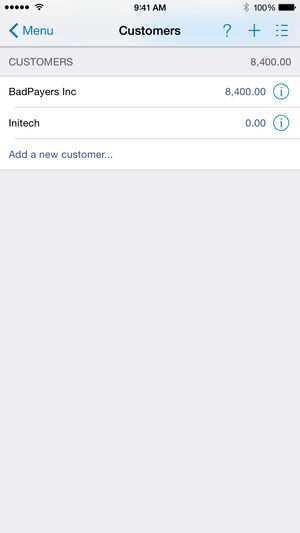The screenshot displays a smartphone's screen interface. At the top, there is a gray border with a hint of blue on the right side. In the top-left corner, there are five black dots adjacent to a Wi-Fi signal icon. Following these, to the right, is the time displayed as 9:41 AM. On the far-right side of this top section, a fully charged battery icon is visible.

Below the gray border, there is a blue menu bar with the word "Customers" in black text centered. To the right of this title, there are three additional icons: a blue question mark, a plus sign, and a menu icon consisting of three horizontal lines with blue dots to the left of each line. 

Beneath this, another gray border runs horizontally, marked with "Customers" on the left and the number "8,400" on the right. 

The main white section of the screen is divided into two parts. The first section lists "Bad Players Inc." with a count of "8,400" on the right side and a blue circle featuring a blue eye icon. Below this, "Inateck" is listed with "0" to the right and a similar blue circle with a blue eye icon. Following these entries, there is an option labeled "Add a new customer..." which suggests the potential to input additional entries.

At the very bottom of the screen, a large gray rectangle stretches to the bottom of the image, completing the layout of the interface.